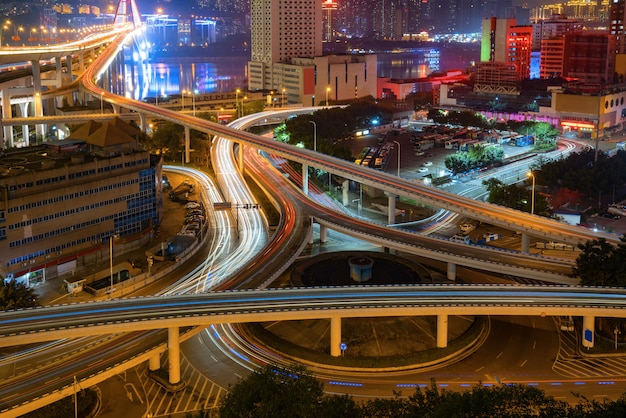This captivating nighttime aerial photograph showcases an intricate interstate system weaving through a bustling, expansive city. In the forefront, an array of highways and streets form a complex network, their paths illuminated by the time-lapsed streaks of car headlights creating continuous, flowing streams of light. Amidst the roads, a rail line—potentially for trains or subway cars—can be discerned, adding to the multifaceted transportation grid.

The cityscape is dotted with a mix of tall buildings and parking garages, a testament to the urban density. Streetlights bathe the scene in a warm glow, complemented by the vibrant city lights that refuse to let the night dim their brilliance. In the background, particularly to the upper right, well-lit parking lots and the neon marquees of various stores stand out, casting colorful reflections around them.

A cluster of buildings, strikingly lit in red, catches the eye, although the source of the illumination remains a mystery, adding an element of intrigue to the scene. In the distance, the faint outline of a large river is visible, providing a scenic backdrop to the urban sprawl. This photograph not only captures the complexity and vibrancy of city life after dark but also highlights the seamless blend of natural and artificial elements in a modern metropolis.